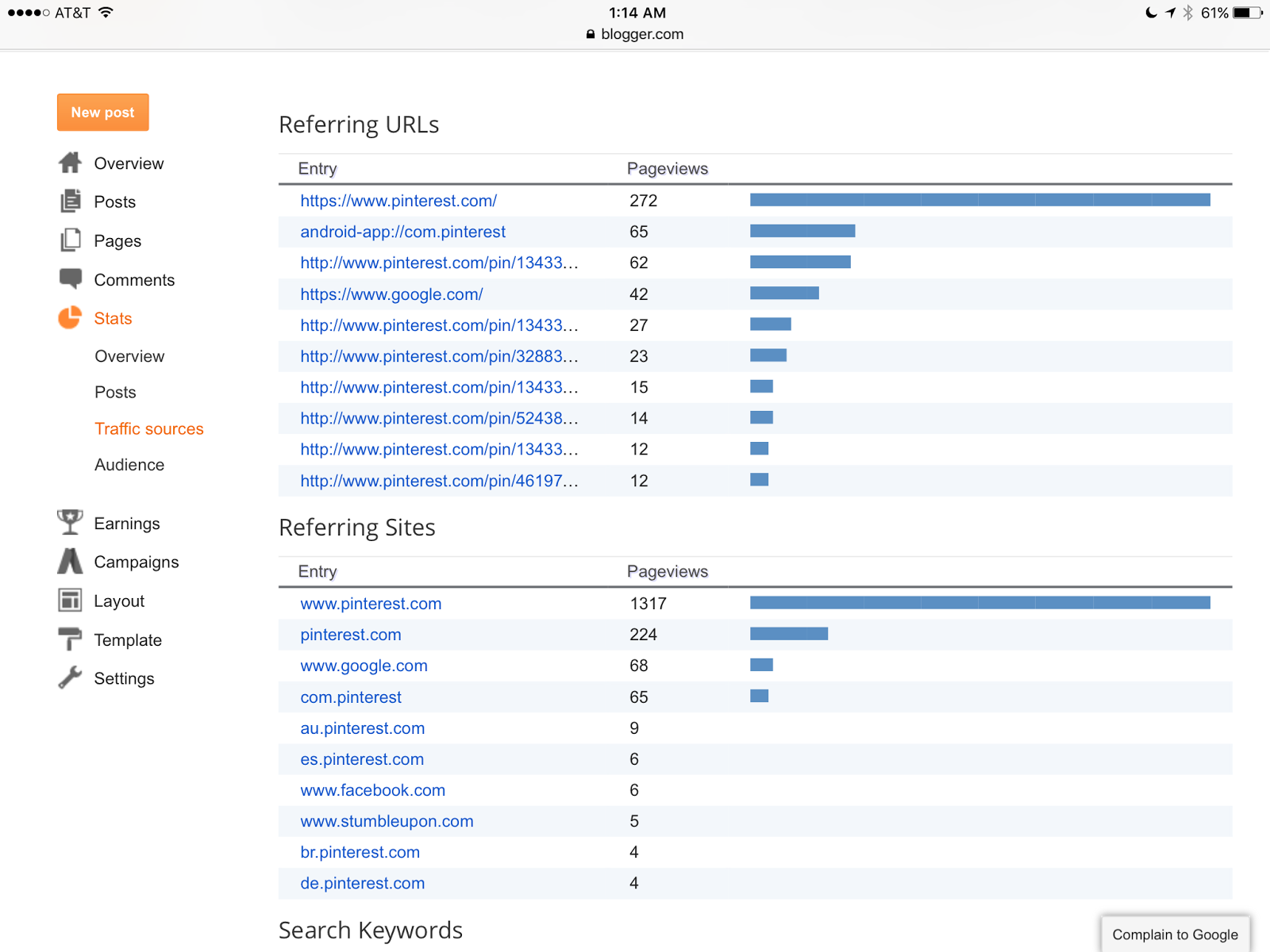This detailed screenshot, taken from blogger.com at 1:14 AM, showcases various interface elements and connectivity indicators on a smartphone, as evidenced by the AT&T network, Wi-Fi connection, 'Do Not Disturb' mode, active location services, Bluetooth, and the 61% battery status visible at the top left corner.

The interface highlights the blog management features of the platform, notably the ability to create new posts and navigate through different sections such as Overview, Posts, Pages, Comments, Stats (which further breaks down into Overview, Posts, Traffic Sources, Audience), Earnings, Campaigns, Layout, Template, and Settings. In this particular screenshot, the 'Traffic Sources' tab is selected.

At the top of the 'Traffic Sources' page, 'Referring URLs' is displayed, detailing a list of URLs that have directed traffic to the blog. The sources include Pinterest.com with 272 page views, Androidapp.com.pinterest with 65 page views, and other variations of Pinterest URLs showcasing different numbers of page views. 

Further down, under the 'Referring Sites' section, Pinterest.com is noted for generating 1,317 page views, with additional versions like au.pinterest.com and es.pinterest.com also contributing varying amounts of traffic. The page also features a 'Search Keywords' section and an option to 'Complain to Google,' providing a comprehensive view of the blog's traffic sources and audience engagement metrics. 

Overall, this screenshot provides a clear and detailed view of the blogger.com interface with specific emphasis on traffic analytics.